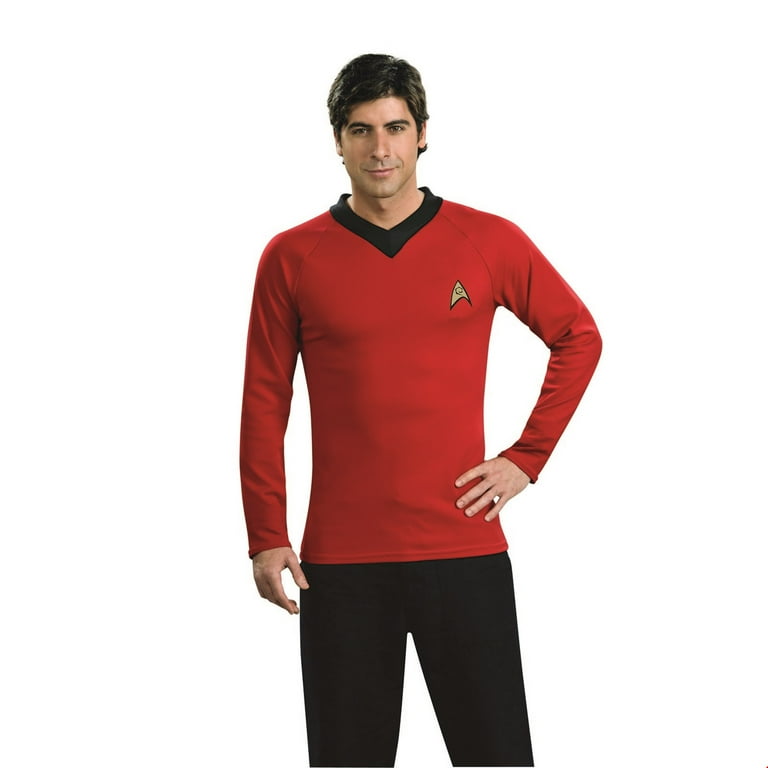A Caucasian man, appearing to be in his late 20s to mid-40s, stands confidently in front of a white background, modeling a classic Star Trek costume. His dark, short-cropped hair complements his clean-cut appearance. He wears a long-sleeved, red shirt with a thick black V-neck collar and matching black trim. On the left side of his chest, there's a distinctive beige insignia resembling a slightly curved triangle with a black border and a small black circle at its center. His attire is completed with black pants, although the material isn't specified. The man's pose is relaxed yet confident, with one arm hanging loose by his side and the other positioned on his hip. He has a pleasant smile on his face, clearly posing for what seems like an advertisement or promotional image. The shot captures him from the knees up, emphasizing the costume's details and fit.